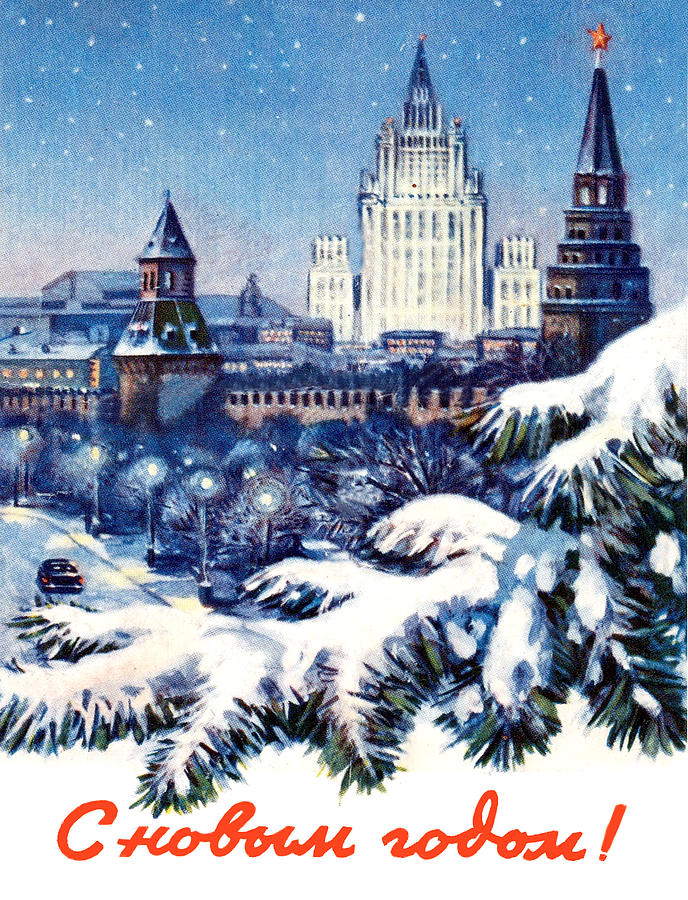The image depicts a computer-animated cityscape at night, blanketed in snow that resembles delicate frosting on green pine tree branches, a scene that evokes the atmosphere of a classic Christmas card. In the foreground, a single pine branch covered in snow adds a touch of depth. A row of five lit street lamps lines the right side of the roadway, illuminating a single old-fashioned brown car with its brake lights glowing. The car is captured driving down a snowy street, adding a feeling of motion and life to the tranquil setting.

At the city's core, a magnificent white building, similar in grandeur to a castle or the Empire State Building but wider, dominates the skyline. Two other prominent city buildings, characterized by their pointed rooftops and darker hues, stand in front of the white structure. Of these, the darker buildings have golden stars adorning their peaks, echoing a festive or regal theme, though one of the smaller dark buildings does not have this decoration.

Snowflakes or stars speckle the dark blue sky, contributing to an almost impressionistic ambiance. The scene includes text in a language unfamiliar to the observers, rendered in elegant red script at the image's bottom, spelling "c-h-o-b-o-w-n-r-o-d-o-m." The visual is detailed and intricate, blending architectural marvels with a serene, snow-covered landscape, encapsulating the quiet, ethereal beauty of a winter night in the city.